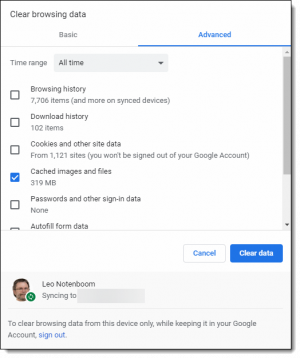This image displays the "Clear Browsing Data" page from a web browser. It shows the "Advanced" settings tab highlighted. The "Time Range" is set to "All Time." Several checkboxes are labeled with data types and the amounts of data stored:

1. **Browsing History:** 7,706 items (plus additional data from synced devices)
2. **Download History:** 102 items
3. **Cookies and Other Site Data:** 1,121 sites (note that clearing this will not sign you out of your Google account)
4. **Cached Images and Files:** 3.9 MB
5. **Passwords and Other Sign-In Data:** None
6. **Autofill Form Data:** No data shown

At the bottom, there are options to "Cancel" or "Clear Data." There is also a profile named "Leo Notenboom" visible, showing that syncing is enabled. The image further suggests that to clear browsing data only from this device while keeping it in your Google account, one must sign out.